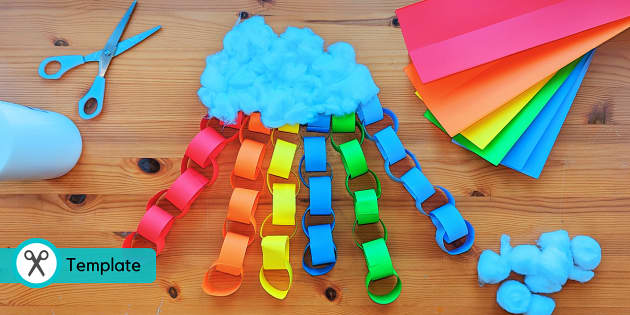The image is a top-down view of various art supplies laid out on the wooden surface of a table, resembling a picnic table. In the top left corner, there is a pair of slightly opened blue scissors next to a white bottle, possibly containing glue, and what appears to be a standing candle. The center of the image features a decorative craft made of colorful paper chains, each loop linked together to form a vibrant rainbow. The chain colors, from left to right, are pink, orange, blue, yellow, green, and blue, with white cotton balls attached to the top, resembling clouds. Additional cotton balls are scattered in the bottom right corner. Situated in the top right, there are neatly folded strips of paper in the colors pink, orange, yellow, green, and blue. In the bottom left corner, there's a small blue banner with a scissors icon and the word "template" beside it, indicating this is a crafting project. The overall scene appears to be styled for a craft tutorial or project thumbnail.